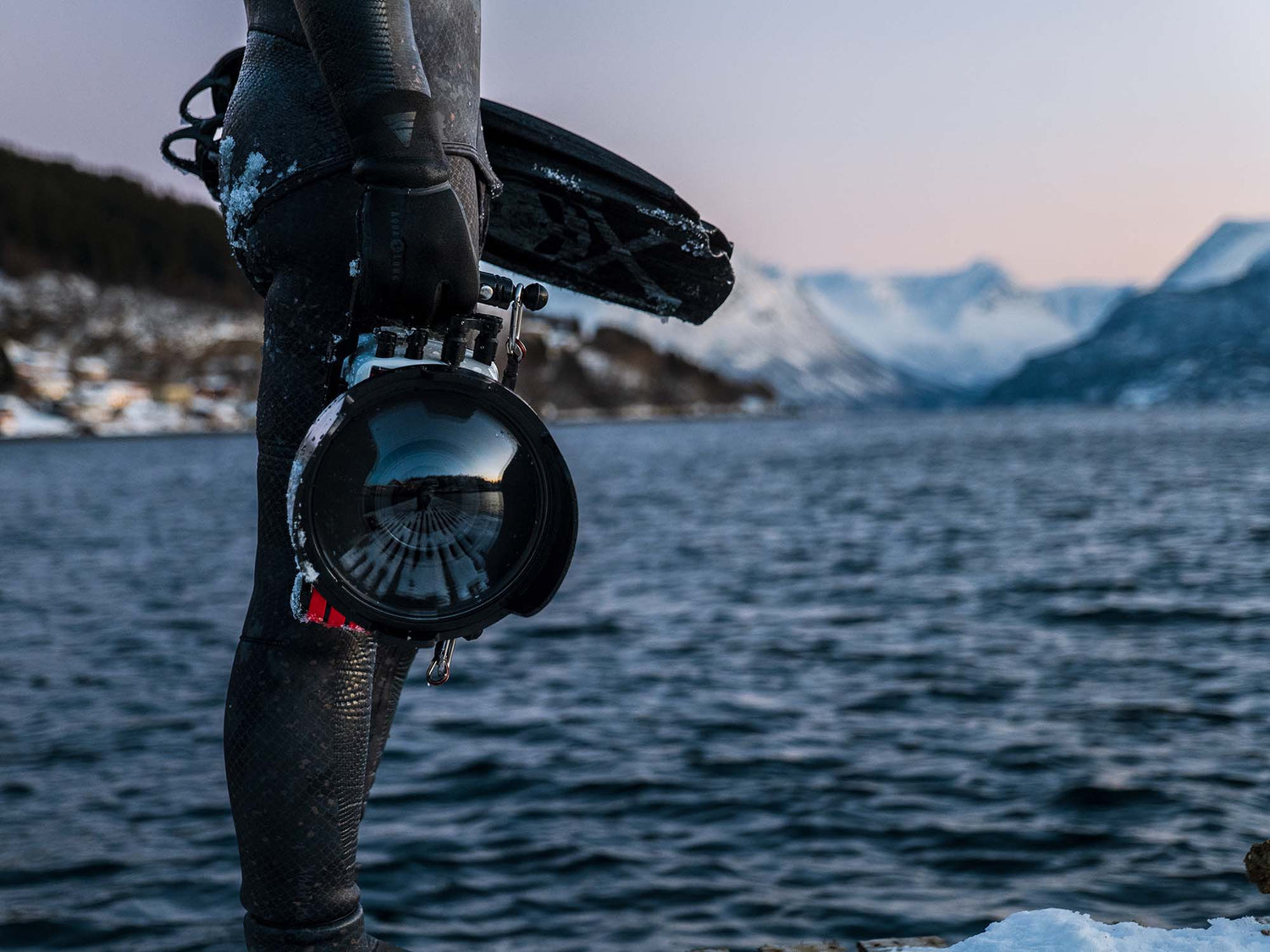This image depicts a diver, clad in an all-black thermal or wetsuit, standing on the icy shore of a fjord or lake nestled between towering, snow-capped mountains. The photograph focuses on the lower half of the diver's body, from the torso down to the ankles, and captures the serene expanse of water stretching towards a distant shoreline, which rises into a picturesque mountain range. On the left side of the frame, a densely wooded hill can be seen. 

The diver, whose build suggests they might be male though obscured by their gear, is holding an enigmatic, sophisticated underwater camera in their gloved right hand, featuring a mirrored oval surface. In their left hand, partially visible behind their profile, they grasp another unidentified piece of equipment. The day is waning under a northern sky painted in hues of orange and purple, yet the sunlight remains diffused and subdued. A sliver of ice and patches of snow are evident at the diver’s feet and the snow-speckled seat of their suit, emphasizing the cold, tranquil environment.